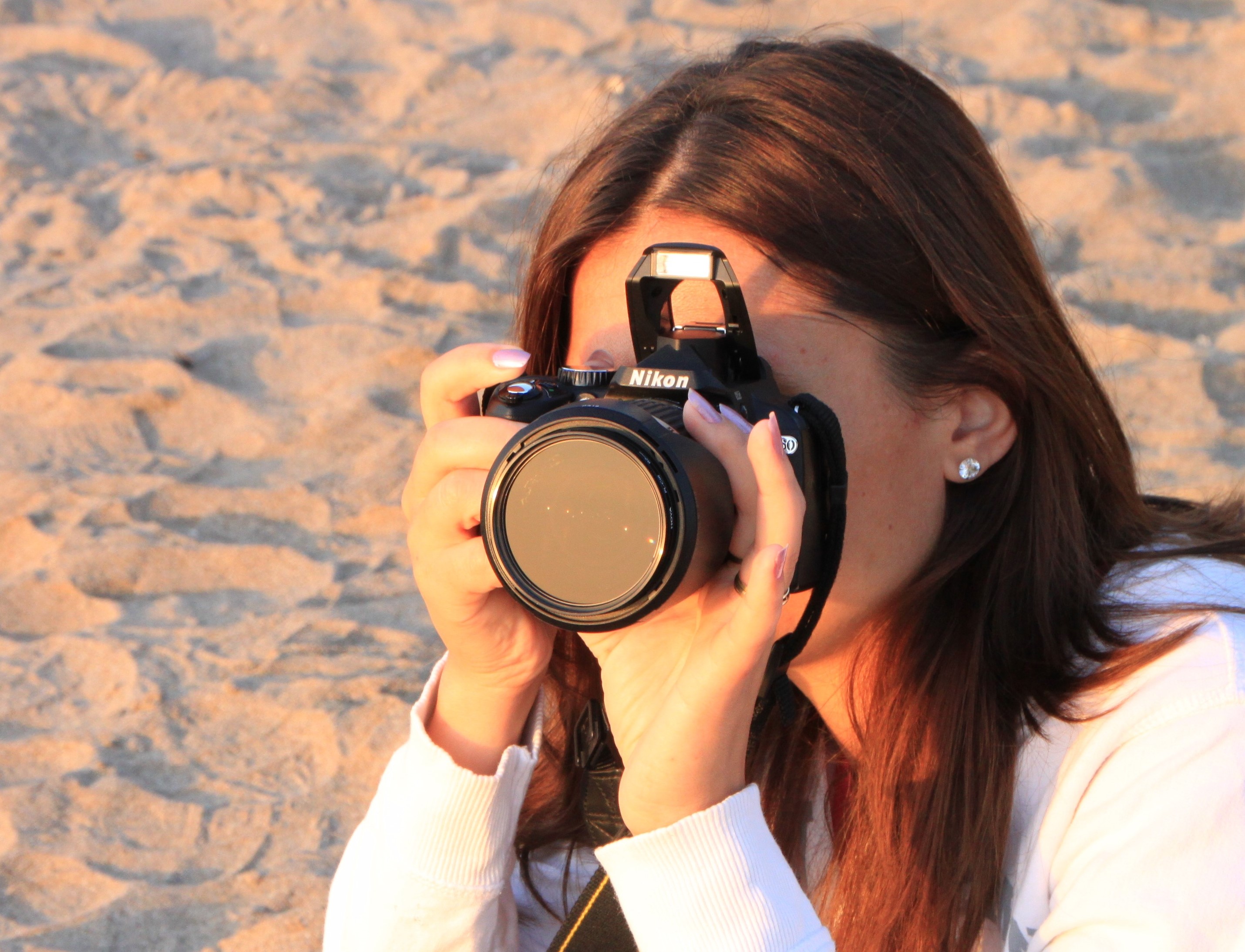In this photograph, a young woman with shoulder-length, brownish-red dyed hair parted in the center is captured in the act of taking a photograph. Her face is obscured by a black Nikon camera with a large, round lens and a flash unit positioned atop. Both her hands grip the camera firmly, revealing her light pink painted fingernails. She is dressed in a white long-sleeved hoodie with the hood down, and her ears are adorned with large yellow gemstone earrings, though one description mentioned small diamond studs. A black camera strap with yellow stitching hangs down in front of her. The right side of her arm is slightly cropped out of the frame. The background features sandy dunes, indicating she is likely in a beach setting. Despite the lens cover being on the camera, she appears engrossed in her photographic endeavor.